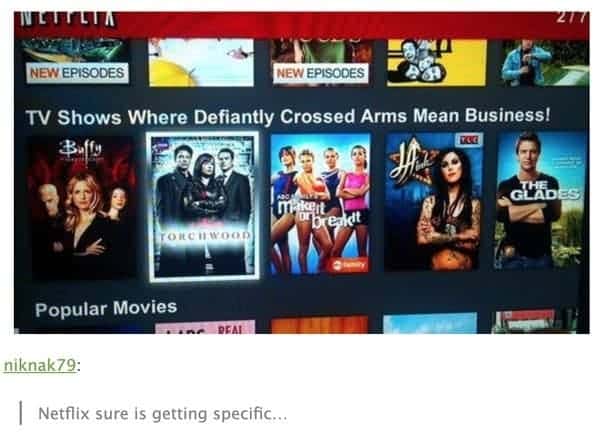Here's the cleaned-up and detailed caption for the image:

---

A screenshot of an older Netflix user interface captures a humorous and oddly specific category curated by the platform. At the top, a red bar displaying the Netflix logo occupies the upper left corner. Below, the category heading reads, "TV shows where defiantly crossed arms mean business," accompanied by images of five different shows. The featured shows include "Buffy the Vampire Slayer," "Torchwood," "Make it or Break it," "LA Ink," and "The Glades," each displaying characters with serious expressions and crossed arms. Beneath this section, a partially visible category labeled "popular movies" peeks through, and the bottom of another category can be seen above. The interface is set against a gray background, with category titles in white text. The Tumblr user NickNackNIKNAK79 humorously comments on the specificity of the category, noting, "Netflix sure is getting specific."

---